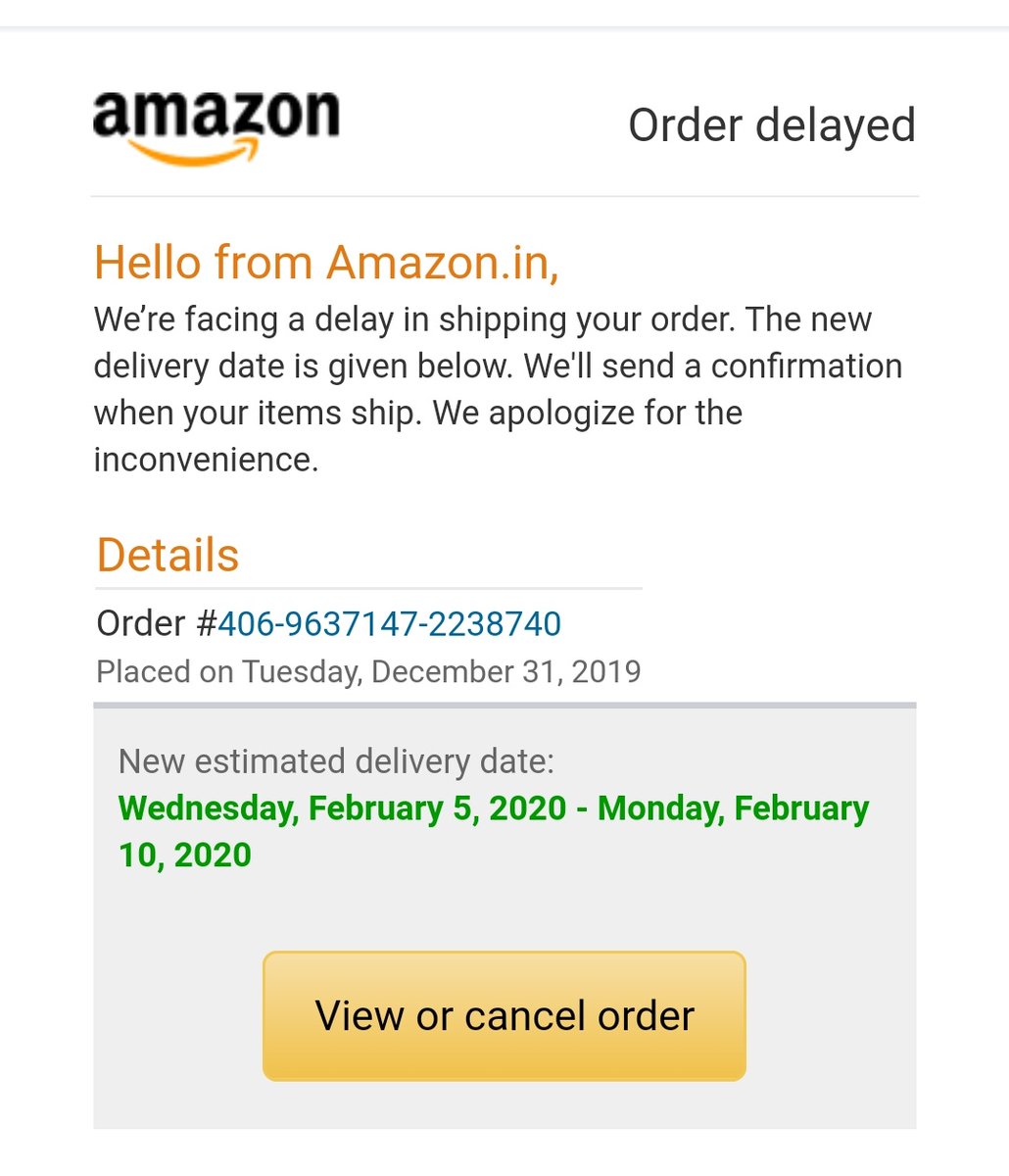The image displays a notification from Amazon regarding an order delay. On the left side of the notification is the Amazon logo, while to the right, the bold text "Order Delayed" is prominently displayed. Below this heading, there is a detailed message outlined in goldish-orange text, which reads:

"Hello from Amazon.in, we're facing a delay in shipping your order. The new delivery date is given below. We'll send a confirmation when your items ship. We apologize for the inconvenience."

Further details of the order are provided, including the order number in blue and the original placement date, which was Tuesday, December 31st, 2019. The new estimated delivery window, shown in green, is from Wednesday, February 5th, 2020 to Monday, February 10th, 2020. At the bottom of the notification, there are options to "View" or "Cancel" the order.